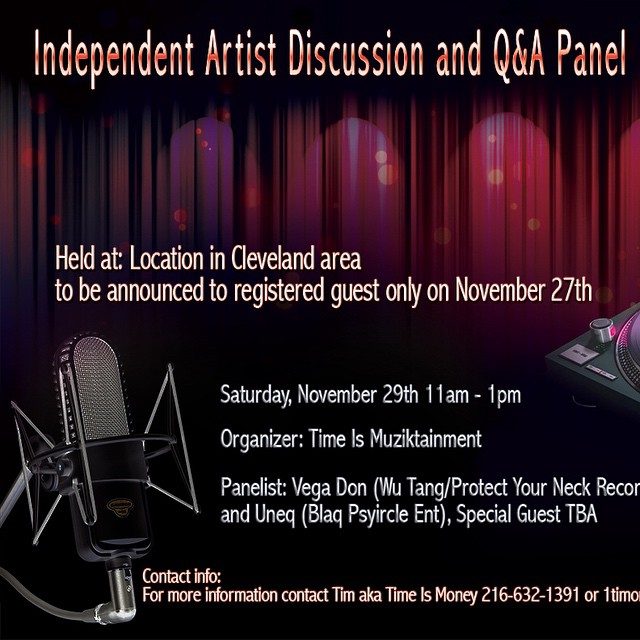This image features the left half of a promotional flyer for an event. At the top, in bold, light-colored font against a black background with an orange gradient and a wavy, sparkly red curtain design, it reads "Independent Artist Discussion and Q&A Panel." The flyer details that the event will be held at a location in the Cleveland area, to be announced to registered guests only, on November 27th. Following this, the date and time are noted: "Saturday, November 29th, 11 a.m. to 1 p.m." The organizer is listed as "Time & Musictainment," and panelists include "Vegadan (Wu-Tang / Protect Your Neck Records)" and "Unique Black Circle Entertainment," with a special guest to be announced. At the bottom, partially cropped off, there are additional details, alongside contact information. A recording studio microphone and a cropped turntable contribute to the flyer’s creative design.